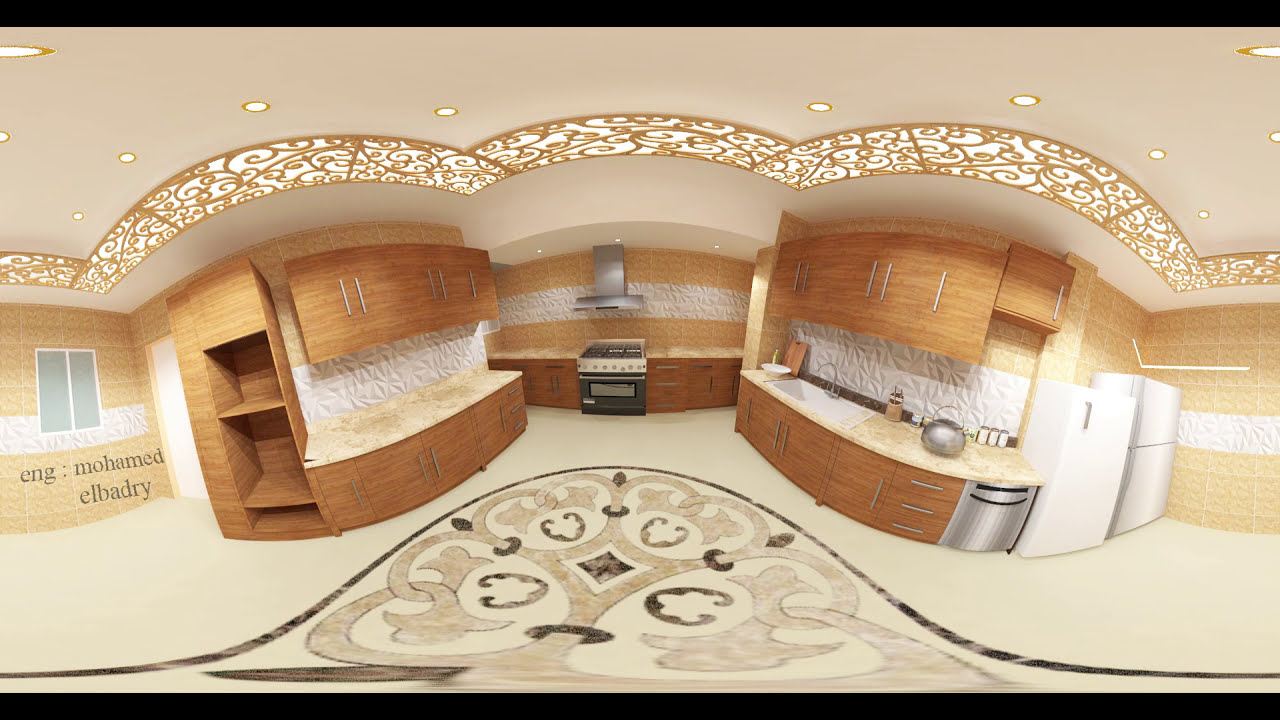This detailed photograph captures the stylish interior of a kitchen, emphasizing its elegant and intricate design. The ceiling showcases a white backdrop adorned with elaborate tan and white archways that cross above both the cabinets and the stove area. The room's walls are lined with brown wood-trimmed cabinets, both lower and upper. These cabinets span the middle left and right of the image, with an identical setup on both sides except for a stainless steel dishwasher on the right. 

The backsplash is a pristine white tile, complementing the white and tan marble tabletops. Central to the kitchen is a sleek stainless steel stove, topped with a matching vent hood. A stainless steel sink and silver tea kettle are also notable features, along with a white refrigerator-freezer combo. The floor is a striking white with an intricate black-and-white arched tile mosaic pattern, featuring classical gray swirls and black diamond motifs. 

Small, round lights are installed across the ceiling, illuminating the room brightly and evenly. Additionally, a set of windows on the left wall display the words "ENG...Mohammed Arbitrary," written in black letters. The panoramic angle of the image subtly distorts the layout but captures the room's spacious and luminous ambiance.